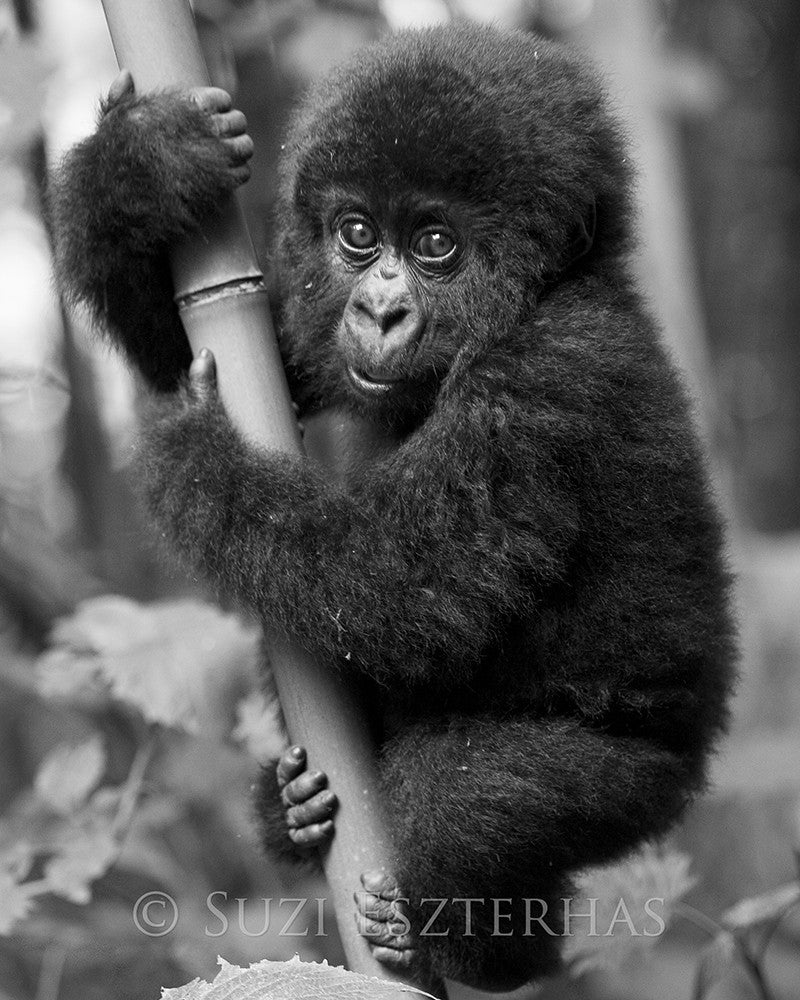In a captivating black and white photograph likely taken at a zoo, a fuzzy baby monkey, possibly a chimpanzee, clings tightly to a bamboo stalk with its small, delicate arms and feet. The young primate, covered in thick, teddy bear-like fur, gazes almost directly at the viewer with its large, expressive black eyes and distinct monkey nose. Behind the monkey, leaves are faintly visible, adding a natural backdrop to the scene. At the bottom of the image, in faded white uppercase letters, is the photographer’s name: Suzi Eszterhas, accompanied by a copyright symbol.